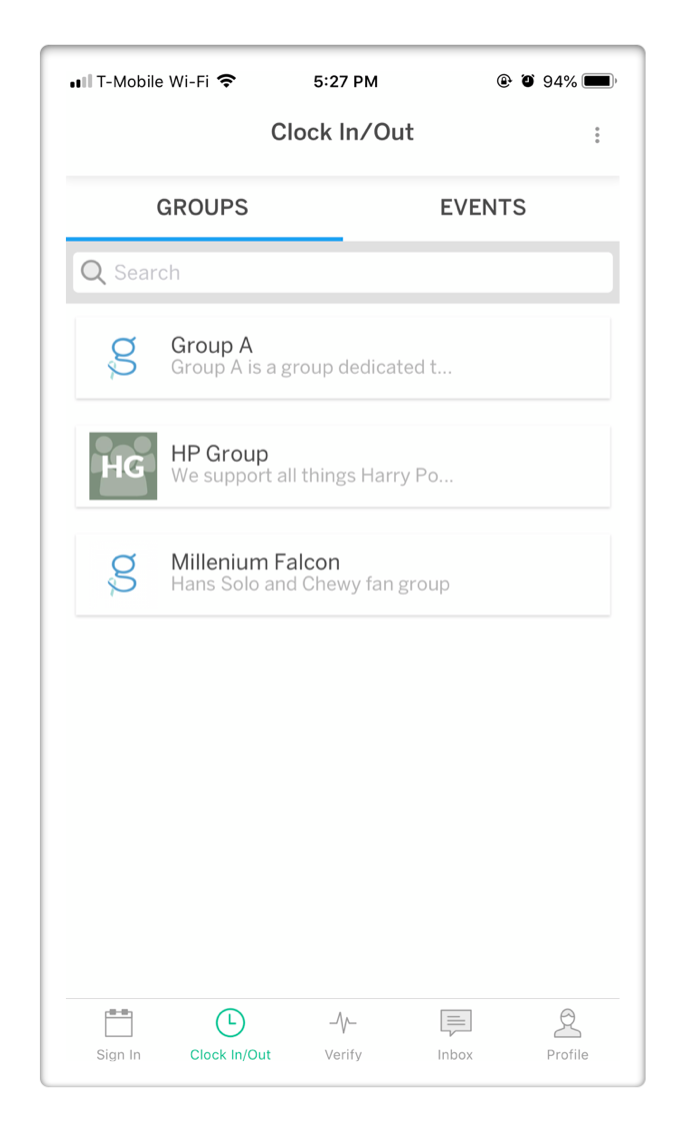The image depicts a mobile phone screen showcasing the interface of a social networking app. At the top, the status bar displays "T-Mobile Wi-Fi," along with Wi-Fi signal indicators, phone service bars, an alarm clock icon, and a battery status showing 94%. Below the status bar, the screen features options for "Clock In/Out," followed by two main tabs: "Groups" and "Events," with the "Groups" tab currently active, indicated by a blue underline.

Under the tabs, there is a search bar followed by a list of groups. The first group, labeled "Group A," contains a partially visible description that reads, "Group A is a group dedicated to..." but the full details remain hidden. The second group, named "HGHB Group," appears to be a community for Harry Potter enthusiasts, despite some ambiguity with the abbreviation "HG." The third group is identified as the "Millennium Falcon group," presumably focused on fans of Star Wars, Han Solo, and Chewbacca.

The interface suggests that these groups are perhaps chat forums or discussion boards where members can engage in conversations related to their respective interests. The "Events" section adjacent to "Groups" is visible but is not currently selected, leaving its contents undisclosed.